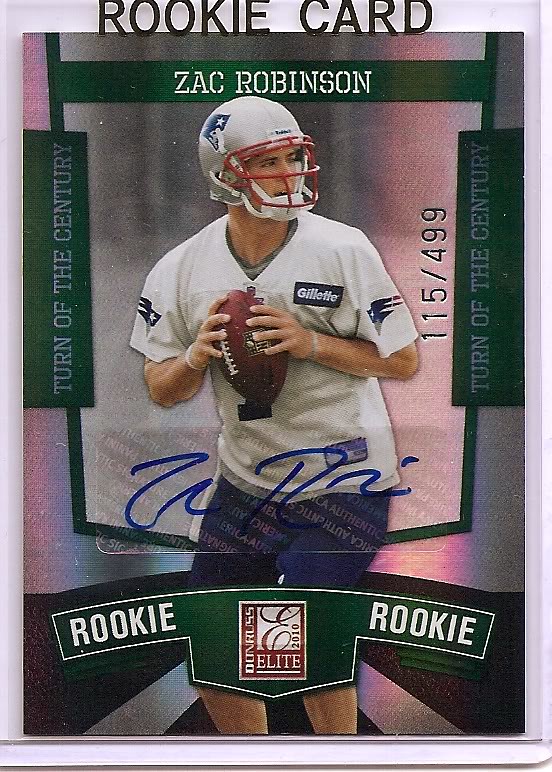This image is of a rookie football card featuring New England Patriots player Zach Robinson. The top of the card prominently displays the text "Rookie Card" above Zach Robinson's name. The photograph on the card shows Robinson in a white short-sleeved Patriots jersey, blue shorts, and a Patriots helmet, holding a football as if preparing to throw it. Surrounding his image, both to the left and right, are the words "Turn of the Century," with the right side including the numbering "115-499." His autograph in blue ink is located around his waistline. At knee level, the word "Rookie" is repeated twice, flanking the "Elite 2010" logo in the center. The card captures his practice setting, likely indicated by the absence of full pads and the presence of a sponsor's logo, specifically Gillette, on his shirt.